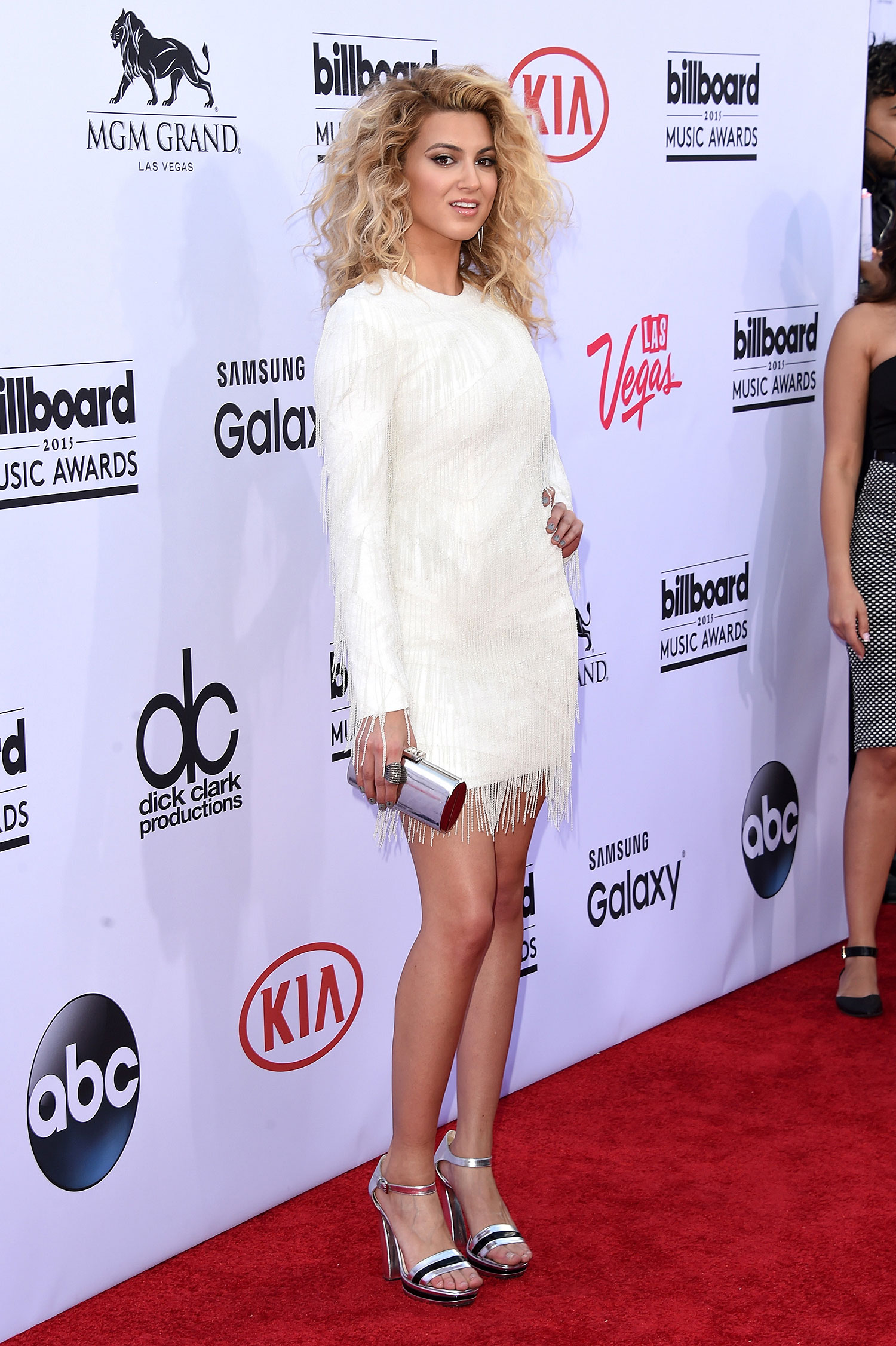In this classic red carpet photo, a young Caucasian woman in her early 20s stands elegantly on a red carpet in front of a logo wall, poised for the camera. She has long, voluminous curly blonde hair that frames her fair-skinned face and cascades over her shoulders. She is dressed in a stylish white long-sleeve mini dress with a rounded collar. The hem of the dress falls at the upper part of her thighs, adorned with white fringe that hangs delicately. She accessorizes her outfit with silver and black high-heeled sandals and clutches a small silver purse with black trim in her right hand, which coordinates with her footwear. Her left arm is bent, with her hand resting on her hip, while her right arm hangs by her side holding the clutch.

The backdrop features a pattern of logos, including those for MGM Grand, Billboard, Dick Clark Productions, ABC, Samsung Galaxy, and Kia, repeating in four rows. The logos are mostly in black with the Billboard and Kia logos repeating in the pattern, the latter in red within a red outlined circle. The wall also contains the event details such as "Music Awards 2015" and "Las Vegas." At the far right of the image stands another woman, partially cut off, dressed in a black strapless top, a gray skirt, and black shoes, suggesting the presence of other attendees at the event. The young woman in focus exudes confidence and grace, fully embodying the glitz and glamour of a red carpet affair.